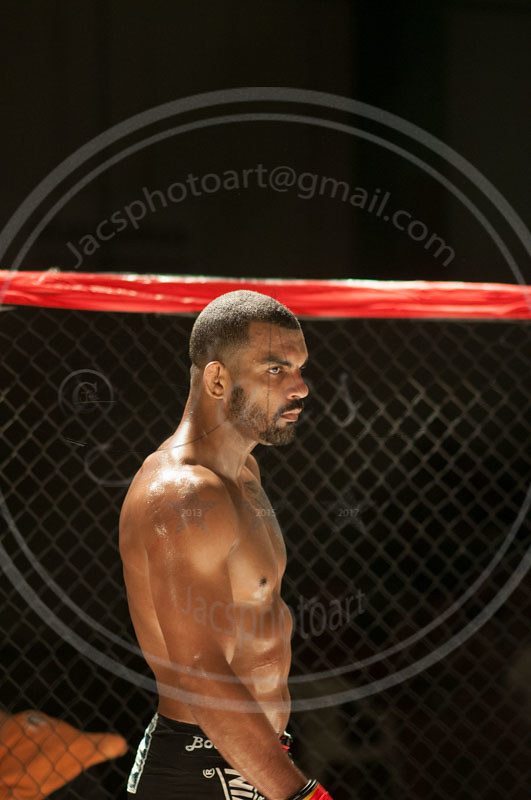The photograph captures a muscular, shirtless man with short dark hair, a well-kept beard, and a mustache. He is glistening with sweat and looking to the right in a profile view. A tattoo of a star adorns his right shoulder. He is wearing black boxing shorts with white, unreadable lettering on the sides and appears to be donning red gloves, though only his wrists are visible. The man is standing in front of what seems to be a chain-link fence, possibly indicating a ring or cage. Extending horizontally at the top of the image is a red line or tarp, suggesting the top boundary of the structure behind him. The background is pitch black, enhancing the faint, superimposed watermark that reads "jacksphotoart@gmail.com" within a transparent gray circle.